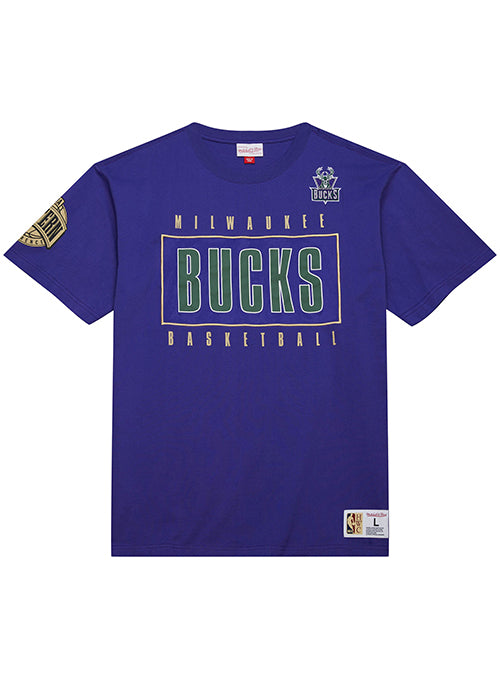Displayed is a Milwaukee Bucks basketball t-shirt lying flat against a pristine white background. The t-shirt features a vibrant cobalt blueish-purple hue. Prominently centered on the front, the word "Milwaukee" is styled in light yellow font, encircling a green box with "Bucks" in large, bold green letters, immediately below which the word "Basketball" appears, also in light yellow.

Adding to the detail, the right sleeve showcases a gold emblem prominently displaying the letters "ERN" at its center. Positioned at the lower right-hand corner of this short-sleeved t-shirt is a label featuring a silhouette of a basketball player accompanied by the letter "L" in black, indicating the size as large.

Inside the back neck area of the t-shirt, there is an internal label with additional size information marked in red. On the left shoulder area, a contrasting black logo highlights the Bucks emblem, adding an extra touch of team pride to this spirited apparel.